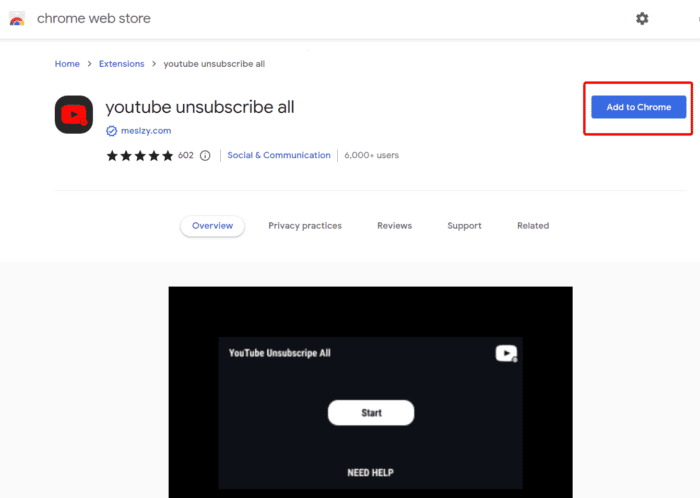This screenshot from the Chrome Web Store showcases the "YouTube Unsubscribe All" extension by MsSizzy.com. At the top, a breadcrumb trail reveals the navigation path: Home > Extensions > YouTube Unsubscribe All. The app's name is prominently displayed alongside its logo, a black square containing a red YouTube icon. It boasts a rating of 4.5 out of 5 stars based on 602 reviews, with an information icon nearby. The extension has been categorized under "Social & Communication" and is used by over 6,000 users.

Four tabs are visible: Overview, Privacy Practices, Reviews, and Support. The Overview tab is highlighted. Below, an embedded YouTube video features a black screen with "YouTube Unsubscribe All" text, a central "Start" button, and "Need Help?" caption. The YouTube logo appears at the top right corner of the video.

In the top right corner of the screenshot, there is a prominent "Add to Chrome" button encapsulated in a red box, encouraging users to install the extension.